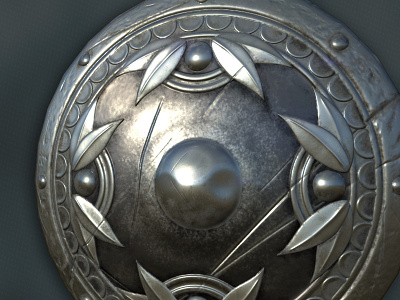This image is a close-up, colored view of a round, silver object, possibly a decorative shield or medallion, though its exact size and context are uncertain. The perimeter of this object is adorned with a smooth band featuring small, button-like protuberances, with at least eight visible around the edge. Surrounding the central area is a ring decorated with half-circle arches. The middle portion is a solid, slightly bulging dark gray surface with a round, nipple-like protrusion in the very center. Positioned at the north, south, east, and west points of this central area are smaller, olive-like shapes, each flanked by two silver leaves angled toward the protrusion. The object, which appears three-dimensional, shows a more pronounced shine on the left side due to the light source, while the background is a dark gray, which further accentuates the silvery sheen of the item.